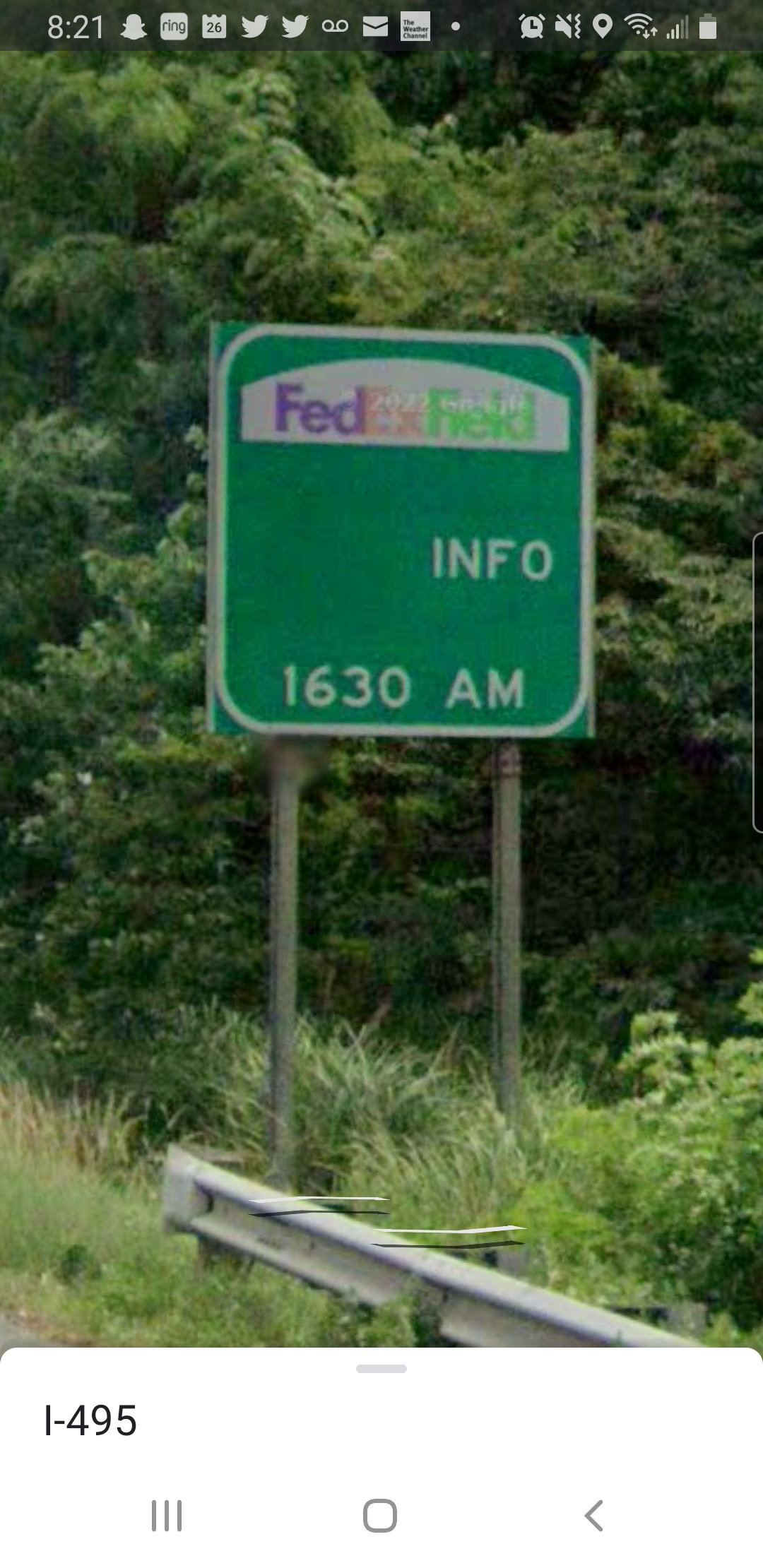A smartphone screenshot capturing a dark green, square-shaped highway information sign on I-495, likely sourced from Google Maps. The top of the sign features a FedEx logo adorned in purple, pink, and bright green on a white background. Beneath the logo, the sign reads “info” in white, followed by “1630 AM,” also in white. The upper part of the screenshot includes typical smartphone interface elements: the time displayed as 8:21, a series of notifications including Twitter alerts, a voicemail, and a new email. The right side of the screen shows the signal strength bars and battery level. The surrounding environment is forested, with visible tall grasses, bushes, and trees in the background.